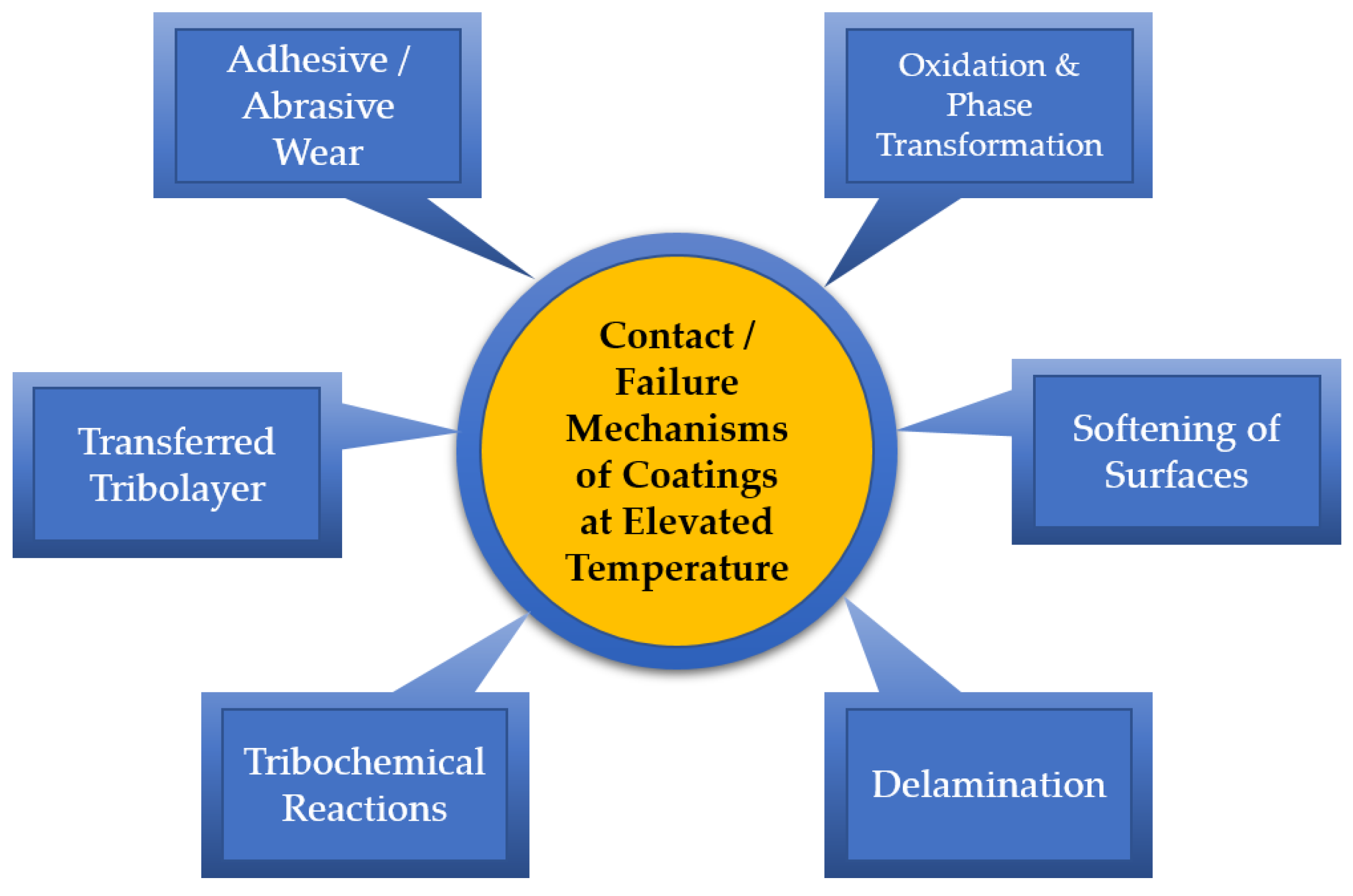This is a detailed illustration presented on a white background, likely created using software like Microsoft PowerPoint. At the center of the graphic, there is a filled gold-colored circle, outlined in blue, containing the black-printed title: "Contact/Failure Mechanisms of Coatings at Elevated Temperature." Radiating outward from this central circle are six rectangular text boxes, arranged around the circle at positions reminiscent of a clock: approximately at 1 o'clock, 3 o'clock, 5 o'clock, 7 o'clock, 9 o'clock, and 11 o'clock. These text boxes, featuring a blue background with white text, list various mechanisms as follows, from left to right starting at the top: "Adhesive/Abrasive Wear," "Transferred Tribo Layer," "Tribochemical Reactions," "Oxidation and Phase Transformation," "Softening of Surfaces," and "Delamination." The organized layout and the use of contrasting colors emphasize the different types of failure mechanisms critical for understanding coatings' behavior at elevated temperatures, potentially serving as an informative guide for workplace safety or materials science.